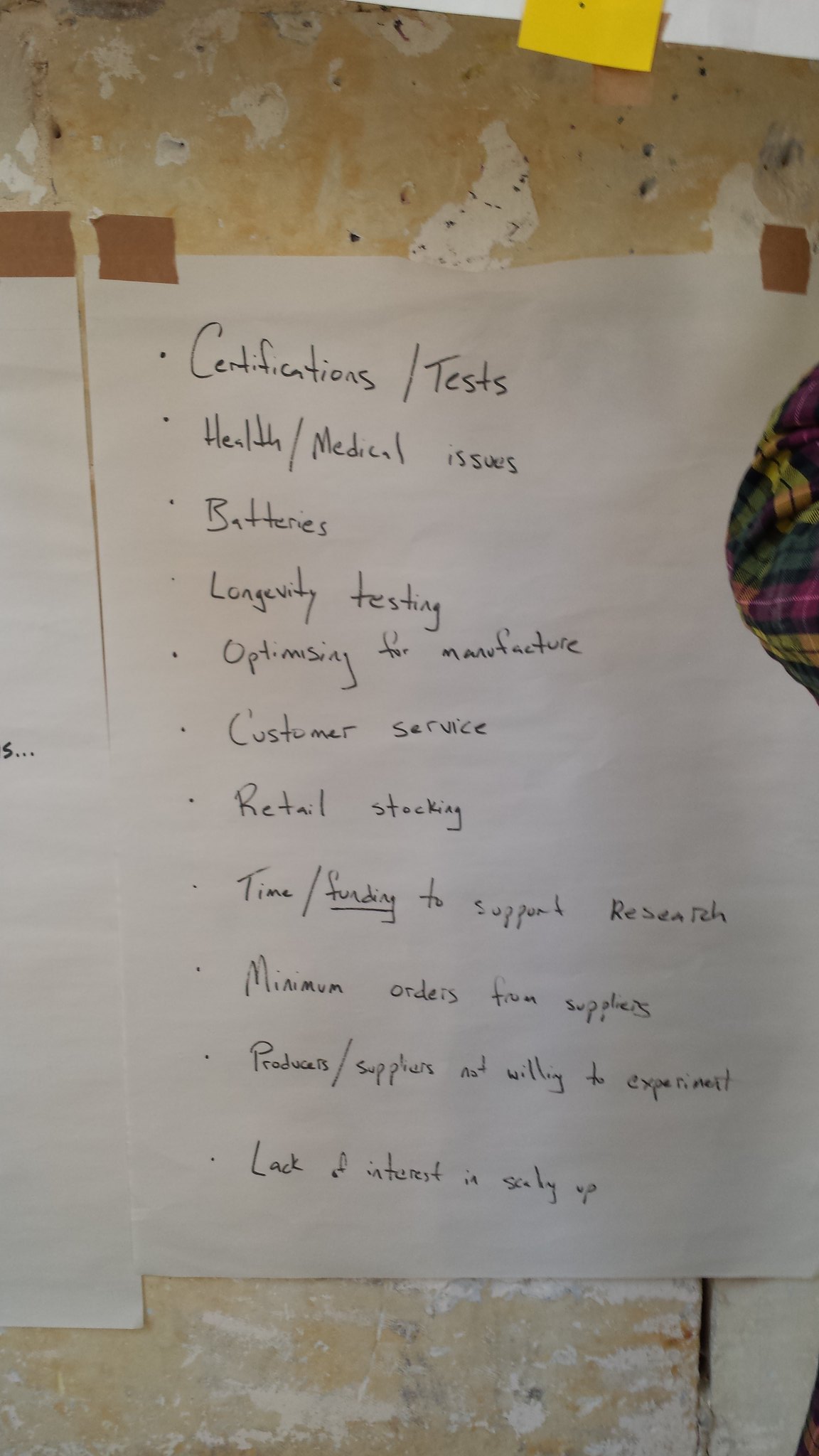The image depicts a handwritten list on plain white paper, affixed with brown tape to a yellow and white spackled wall, possibly a tan-colored bulletin board. The paper is slightly worn, with pinholes indicating previous use. To the right of the list, there's a piece of cloth featuring a vibrant plaid pattern in yellow, green, blue, red, and orange, which might be part of a shirt or a bag. Below the tape, the wall shows some streaks of paint. The list is organized with bullet points running vertically and reads: 

1. **Certification/Tests**
2. **Health/Medical Issues**
3. **Batteries**
4. **Longevity Testing**
5. **Optimizing for Manufacture**
6. **Customer Service**
7. **Retail Stocking**
8. **Time/Funding to Support Research**
9. **Minimum Orders from Suppliers**
10. **Products/Suppliers Not Willing to Experiment**
11. **Lack of Interest in Scaling Up**

Each bullet point is written clearly, highlighting various operational and logistical challenges.